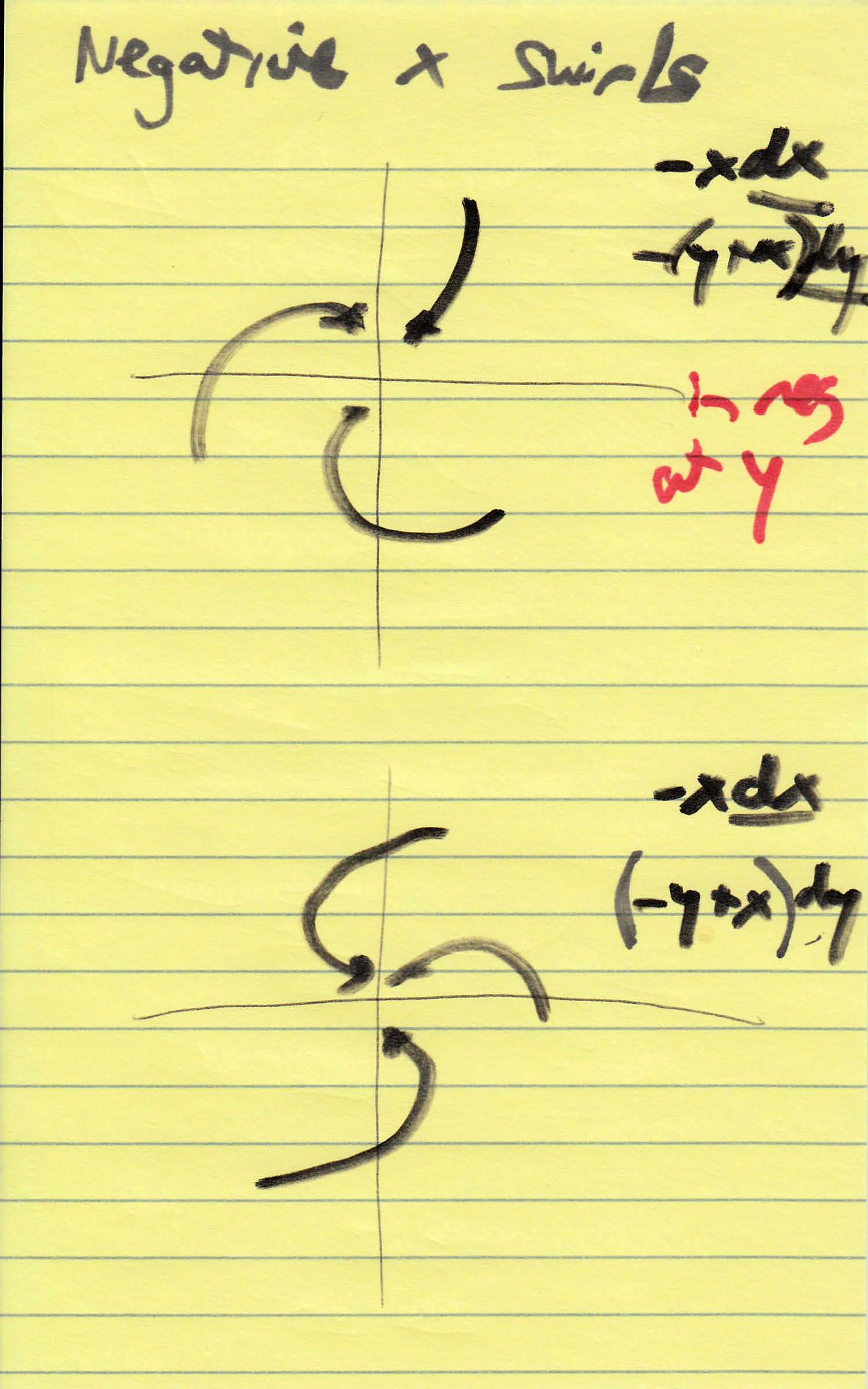The image features a bright yellow sheet of paper with light blue horizontal lines, resembling a standard lined notebook page. On the paper, text and drawings are rendered in black and red marker. At the top, the heading "Negative X Swirls" is written in a combination of regular and cursive handwriting. Below the heading, the page contains several sections of writings and sketches. 

One prominent feature is a graph divided into four quadrants by a cross, with arrows swirling in a clockwise motion around the central intersection. Adjacent to the graph are various letters and equations, also written in both black and red marker, including expressions such as "negative y plus x" and "negative x dx." The handwriting is somewhat messy, yet the equations and annotations are discernible. Additionally, the paper appears to have a few wrinkles, adding a touch of texture to its surface.